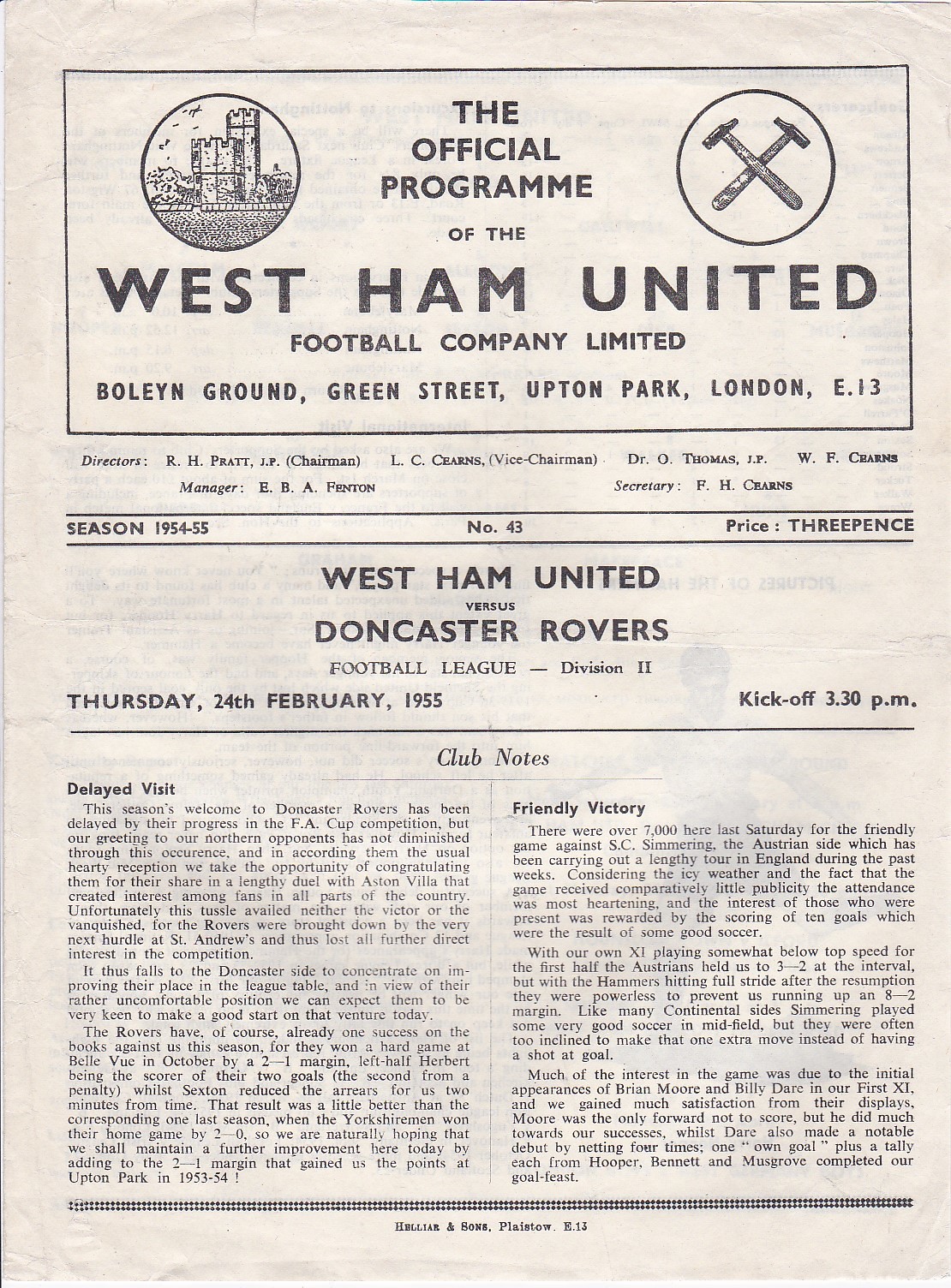This vintage magazine page features the official program of the West Ham United Football Company Limited, dating back to the 1954-55 season. The top section, enclosed in a white rectangle with a thin black outline, prominently displays the club's name alongside its address at Bowling Ground, Green Street, Upton Park, London, E13. Flanking this title are two circular logos: one on the left depicting a castle, and another on the right showing two crossed hammers. Beneath this header, the issue is marked as Number 43 and priced at 3 pence. The program details an upcoming match, West Ham United versus Doncaster Rovers, scheduled for Thursday, 24th February 1955, with a kick-off at 3.30 pm. Accompanying this announcement is a richly detailed article and club notes about the game, spread across two columns, giving readers in-depth insights into the match. The aged, off-white paper adds to its nostalgic charm, being so thin that the text from the opposite side is faintly visible.